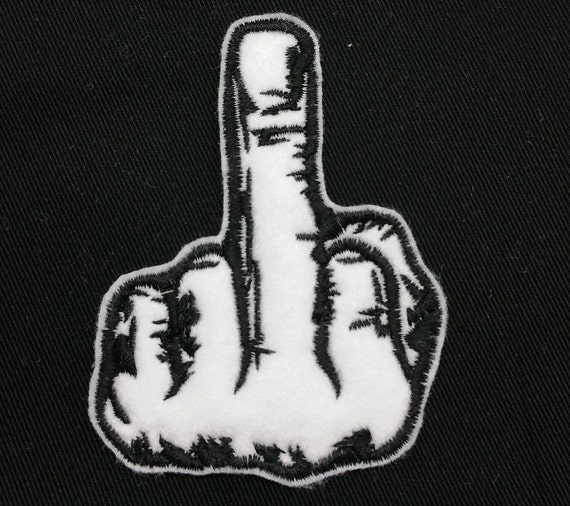The image is a highly detailed black and white drawing, resembling a stitch or sewn design, of a person's left hand prominently giving the middle finger. The hand appears on a black background, possibly representing a black jacket or linen. The hand is predominantly white, with distinct black shadowing accentuating the knuckles, the straight-up middle finger, and the back of the thumb which peeks out from behind. The ring, index, and pinky fingers are curled into a fist, with the knuckles slightly above them and the index knuckle positioned slightly higher. The nail of the middle finger is clear and detailed, showcasing very minimal flesh. Additionally, there is a notable white dot near the top right of the middle finger, adding to the shading effect. The entire depiction is primarily framed within the upper two-thirds of the image, which highlights the intricate contrasts between the white hand and its dark background.